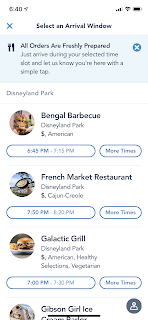This image appears to be a screenshot, likely taken from a smartphone, potentially an Android or iPhone, displaying a mobile application interface. The image is in portrait orientation and quite blurry, making some details challenging to discern. Here's a detailed breakdown of the visible elements:

1. **Top Bar:**
   - A small, indiscernible icon on the left.
   - The number '40' in black text.
   - A triangle icon pointing to the upper right.
   - Standard status icons indicating the signal strength (3 out of 4 bars), Wi-Fi connection, and battery level (approximately 90% full).

2. **Main Header:**
   - On the top left, a blue 'X' icon.
   - Centrally, the text "Select an Arrivals Window," suggesting the selection of a time slot for something, perhaps a food order or reservation.
   - Below, a blue box containing a black fork and knife icon, with text indicating, "All orders are freshly prepared." Below that, the instruction to "Just arrive during your selected time slot and let us know you're here with a simple tap."

3. **Menu Options:**
   - **Option 1:**
     - An unclear circular icon possibly depicting food, potentially a burger.
     - Text: "Bengal Barbecue"
     - Location: "Disneyland Park"
     - Pricing: A single dollar sign ($)
     - Timing: A blue-outlined oval with white interior showing "6:45 p.m. - 9:15 p.m."
     - An additional oval that likely says "More Times."

   - **Option 2:**
     - Circular icon too blurred to identify, possibly a blue sky with something black and white.
     - Text: "French Market Restaurant"
     - Location: "Disneyland Park"
     - Pricing: A single dollar sign ($)
     - Cuisine: "Cajun Cuisine"
     - Timing: Blue-outlined oval with white interior showing "7:50 p.m. - 8:20 p.m." and another oval saying "More Times."

   - **Option 3:**
     - Circular icon showing what looks like a burger and fries on a white plate.
     - Text: "Galactic Grill"
     - Location: "Disneyland Park"
     - Pricing: A single dollar sign ($)
     - Cuisine: "American, Healthy"
     - Food Options: Possibly "Vegetarian Selection"
     - Timing: Blue-outlined oval with white interior showing "7:00 p.m. - 7:30 p.m." and another oval saying "More Times."

   - **Option 4 (Partial View):**
     - Partially visible circular icon, possibly depicting something tan and white like ice cream.
     - Text: "Gibson Grill" followed by "ice" and a thick black bar.
     - Additional text below that is cut off and unreadable.
     - A gray circle with a white person icon is to the upper right of this segment.

This descriptive caption details the entire structure and elements visible within the blurry screenshot, aiming to give a comprehensive understanding of the menu and interface layout shown in the image.